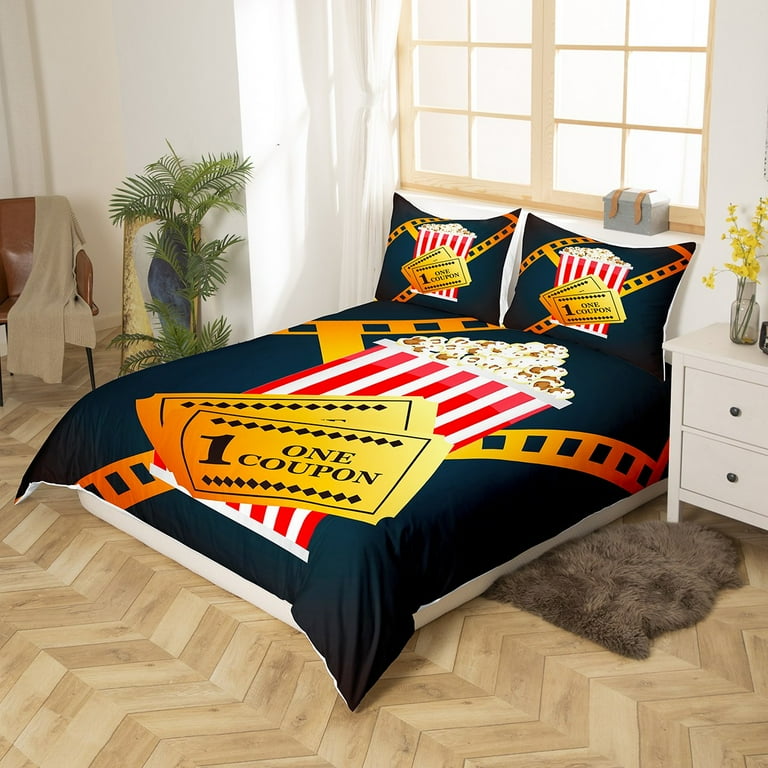This product photo showcases a meticulously designed bedroom. At the center is a bed adorned with a striking black comforter and pillow shams, all featuring a vivid graphic of a red and white striped popcorn bucket brimming with golden yellow popcorn, flanked by two giant golden movie tickets that read "one coupon" in black letters. Additionally, a golden camera film graphic provides a cinematic touch to the bed set. 

The bed is set against a pristine white wall with natural wood-paneled windows that allow natural sunlight to flood the room. These windows complement the light-colored herringbone patterned wood floor beneath the bed. In the middle of the bed, a small gray rug adds a cozy texture. 

To the right of the bed, a small white dresser with two drawers is topped with a vase filled with cheerful yellow flowers. Adjacent to this dresser, a gray fluffy rug lays beneath the right side of the bed, adding further comfort. On the left side, a lush green plant enhances the room’s natural aesthetic. Beside the plant, a brown leather chair with a tan throw blanket draped over it provides a warm, inviting seating area. This detailed and cohesive look creates a perfect blend of comfort and cinematic flair.